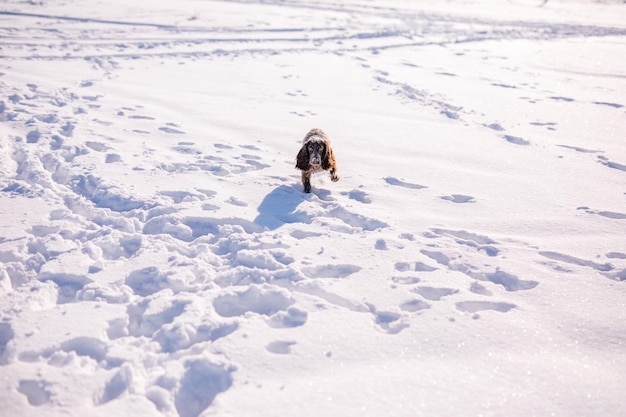The landscape-oriented picture features a bright snowy field crisscrossed with numerous tracks from people, animals, and vehicles. The snow appears to be moderately deep, possibly between six to eight inches. Dominating the scene amidst the vast white expanse is a brown and white dog, energetically running directly towards the camera. The dog, possibly a small breed like a Border Collie, has one foreleg lifted in mid-stride, its droopy ears flapping slightly and a black nose contrasting against its white snout. Its mouth is closed, and small footprints trail behind it, showing its path through the snow. There are no other people or animals in sight, emphasizing the solitary, joyful sprint of the dog against the expansive, treaded snowy landscape.